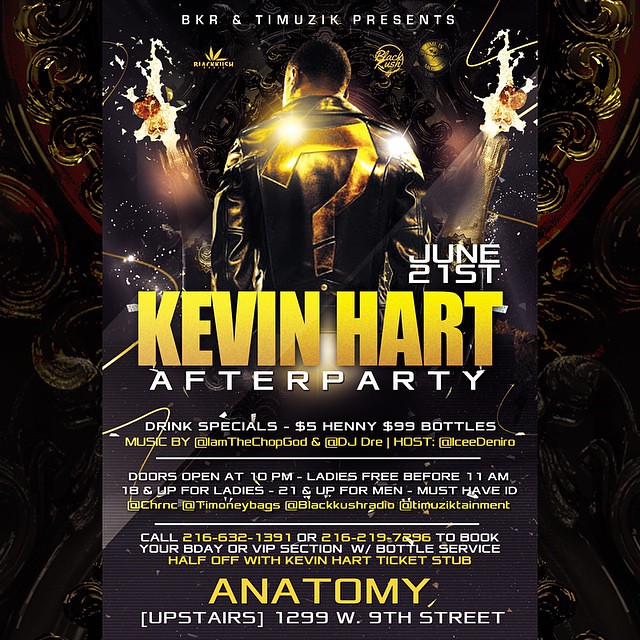This advertisement flyer promotes Kevin Hart's After Party, taking place on June 21st. At the top, white text announces "BKR and Timizik presents." Dominating the flyer is an image of Kevin Hart facing away in a shiny black leather jacket with a large, blocky gold question mark embroidered on the back. The jacket's reflective qualities are enhanced with multiple light reflections. 

In large yellow text, "Kevin Hart" stands out below the image, followed by "After Party" in white text. Above "Hart," the date "June 21st" appears in white. Below "After Party," details about drink specials are listed: $5 Hennessy and $99 bottles. Music will be provided by @IAmTheChopGod and DJ Dre. 

Further information includes hosting by Ice De Niro, noting that doors open at 10 p.m. Ladies enter free before 11 a.m. with age restrictions of 18 and up for ladies and 21 and up for men, requiring ID. The venue, Anatomy, is highlighted in gold text, with the location specified as "upstairs" at 1299 West 9th Street. Social media contacts and phone numbers for more details are also provided, along with small logos on the left and right of the main image.